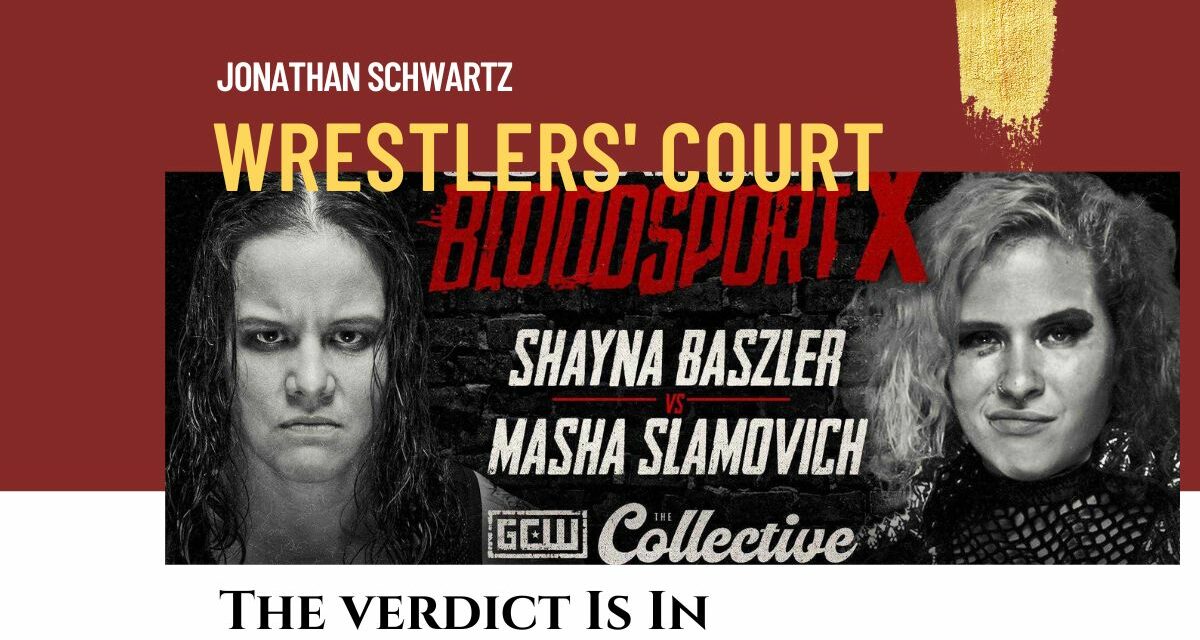This striking advertisement for GCW's The Collective showcases an intense wrestling match with formidable detail. The backdrop features a deep burgundy base with a bold swath of gold paint running across it, adding dramatic flair. Superimposed on this background is a prominent, partially overlaying black-and-white image of two fiercely poised female wrestlers, centered within a black triangular frame. On the left stands a wrestler marked by dark hair and intense dark makeup, and on the right, her opponent boasts lighter, curly hair, a black mesh top, and a confident smirk with a lifted eyebrow.

Text elements add to the excitement and drama: “Jonathan Swartz” is displayed in white against the burgundy background, while “Wrestler's Court” in gold lettering spans both the burgundy and the black-and-white zones. Positioned between the two wrestlers, in bold red text, are the words “Bloodsport X.” Their names, Shayna Baszler and Masha Slamovich, are clearly presented, promising a fierce showdown. This event, hosted by GCW The Collective, is underscored by the tagline beneath the wrestlers: “The verdict is in.”